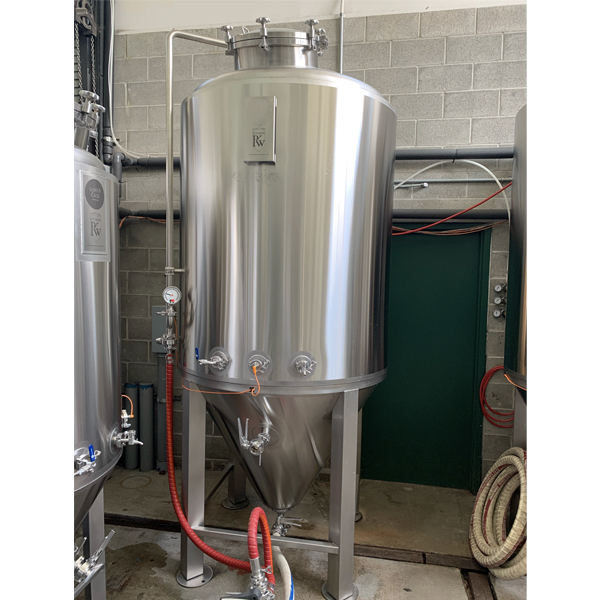In a spacious warehouse, a long, cylindrical machine, likely designed for distillation processes, stands prominently. Its sleek, metallic silver surface gleams under the industrial lighting, suggesting it could be part of an alcohol distillery setup. Though no alcohol bottles are visible, the machinery hints at such a function. An orange cord extends from the middle of the machine, disappearing out of view and contributing to its intricate connections. Additionally, a prominent knob on the machine features a red hose connected to it via a connector resembling a washer, hinting at the complexity and functionality of the equipment.